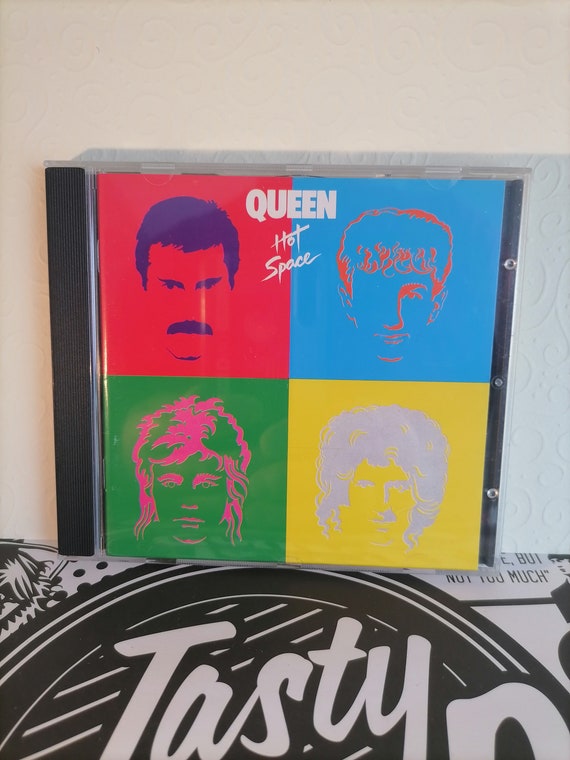This is a vertically oriented photograph featuring a CD case positioned against a white wall, which has some light embossing. The foreground showcases a surface that resembles a table, adorned with a black and white design reminiscent of newspaper print, including black markings and polka dots. Notably, there is a black circle on the table with the word "TASTY" inscribed in white text.

The focal point of the image is a transparent CD case with a black edge on the left, displaying the album "Queen Hot Space." The album cover is divided into four distinct quadrants, each showcasing a band member from Queen in a Warhol-esque, colorful style. The upper left quadrant features Freddie Mercury’s face in purple on a red background. The upper right quadrant displays a band member in an orange silhouette against a blue background. The bottom left quadrant shows another member with a pink silhouette on a green background, while the bottom right quadrant contains a grayish silhouette on a yellow background. Each segment highlights the band members' facial features through colorful line drawings and silhouettes.